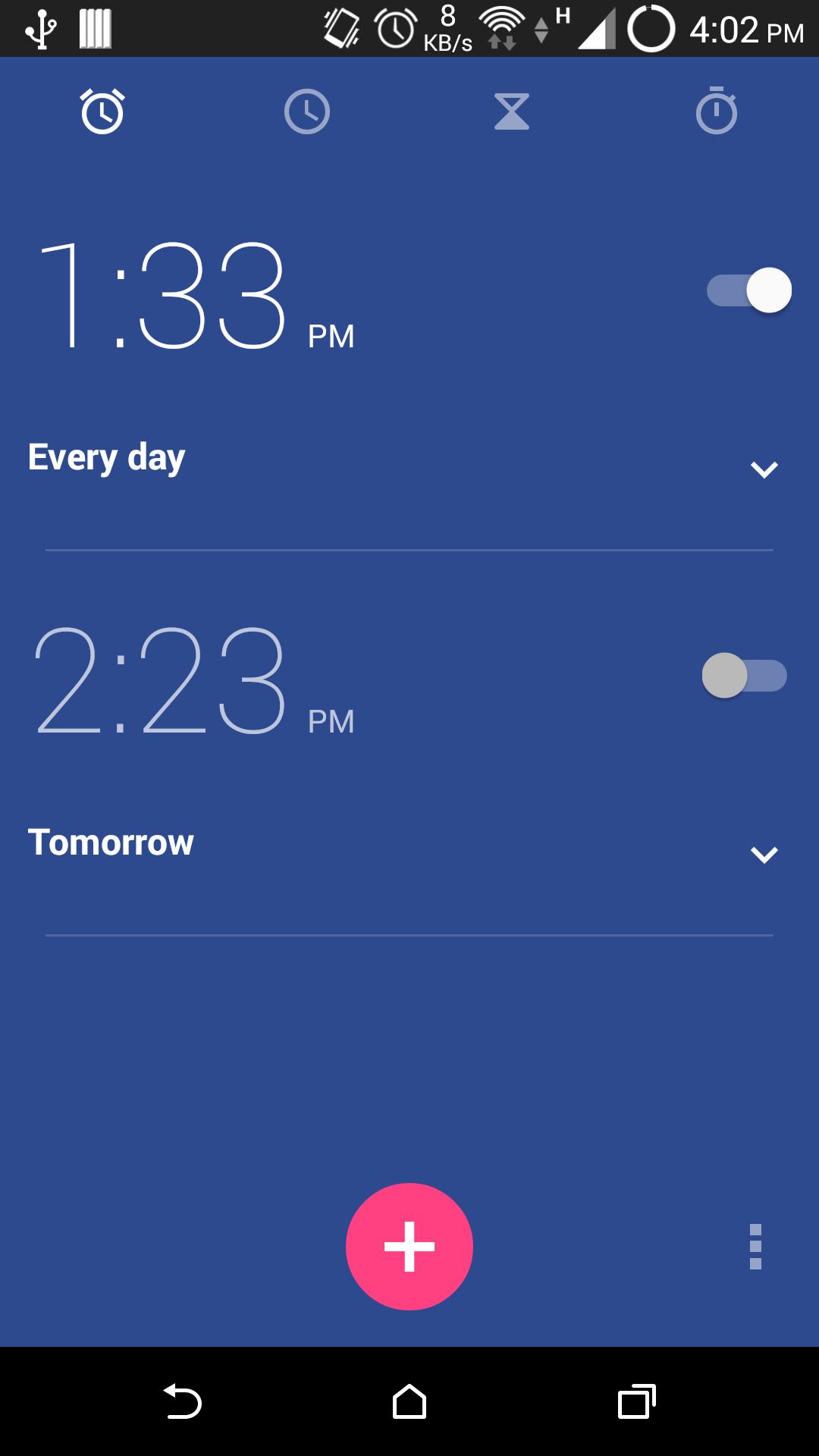The image displays a screenshot of a mobile device showcasing an alarm setting within an alarm app. The interface features two prominent alarms: the first alarm is set for 1:33 PM and is activated to ring every day. The second alarm is scheduled for 2:23 PM but is currently turned off, designated for activation tomorrow. Each alarm entry includes a drop-down menu option for adjusting the timing, although these menus are not expanded in the screenshot.

At the bottom of the screen, there is a conspicuous pink circle containing a white plus symbol, likely for adding new alarms. Adjacent to this circle are three vertically aligned dots, suggesting a settings or additional options menu.

Beneath these elements, a black navigation bar is visible, featuring white icons for back, home, and tabs functions. At the top of the screen, the status bar indicates the time as 4:02 PM, along with symbols for alarm, vibration mode, and internet connection status, all in white text against a black background.

The app's user interface is predominantly navy blue, with various icons representing different time-related functionalities within the app.